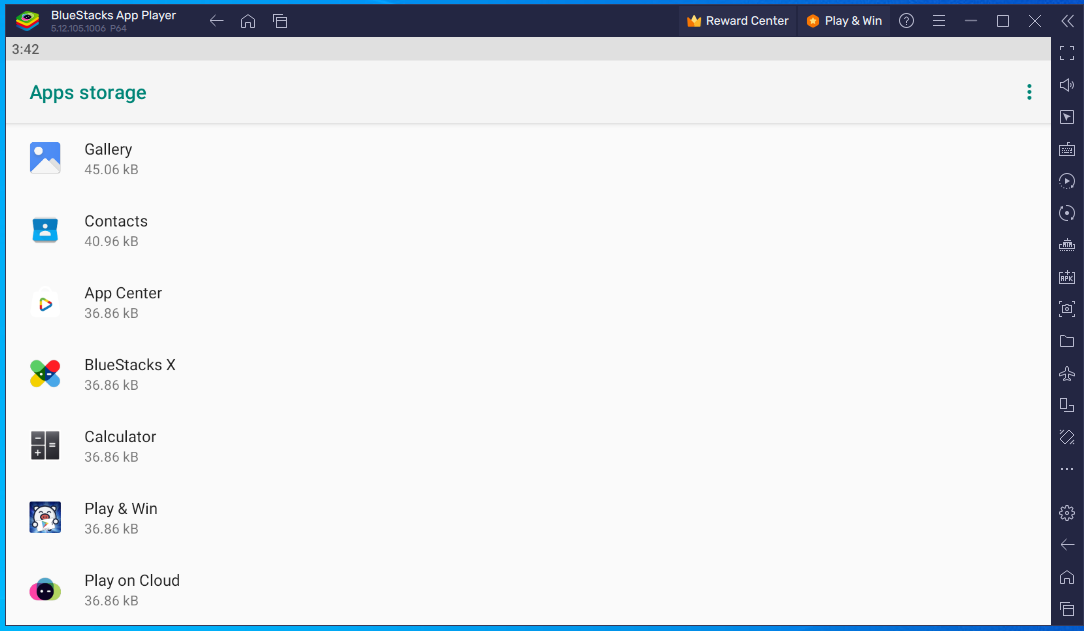The image depicts a webpage showcasing the BlueStacks App Player interface. In the top left corner, there is vibrant artwork featuring a stack of books in various colors: green, yellow, red, and blue. Adjacent to the artwork, the text "BlueStacksAppPlayer" is displayed prominently. Beneath this, the version number "5.12.105.1006 p64" is visible.

To the right of the BlueStacks branding, a series of control buttons is arranged horizontally. These include a back button, a home button, and a tab button. Further to the right, several interactive buttons are visible: one labeled "Rewards Center" accompanied by a crown logo, another labeled "Play and Win," and icons for assistance (question mark), additional options (more icon), minimizing the window (minimize icon), entering full screen (full screen icon), and closing the window (X button icon).

Further down on the left-hand side of the interface, the number "3.42" is displayed, followed by the label "Apps Storage." Below this, there is a grid or list layout showing various app icons available for use or installation within the BlueStacks App Player environment.